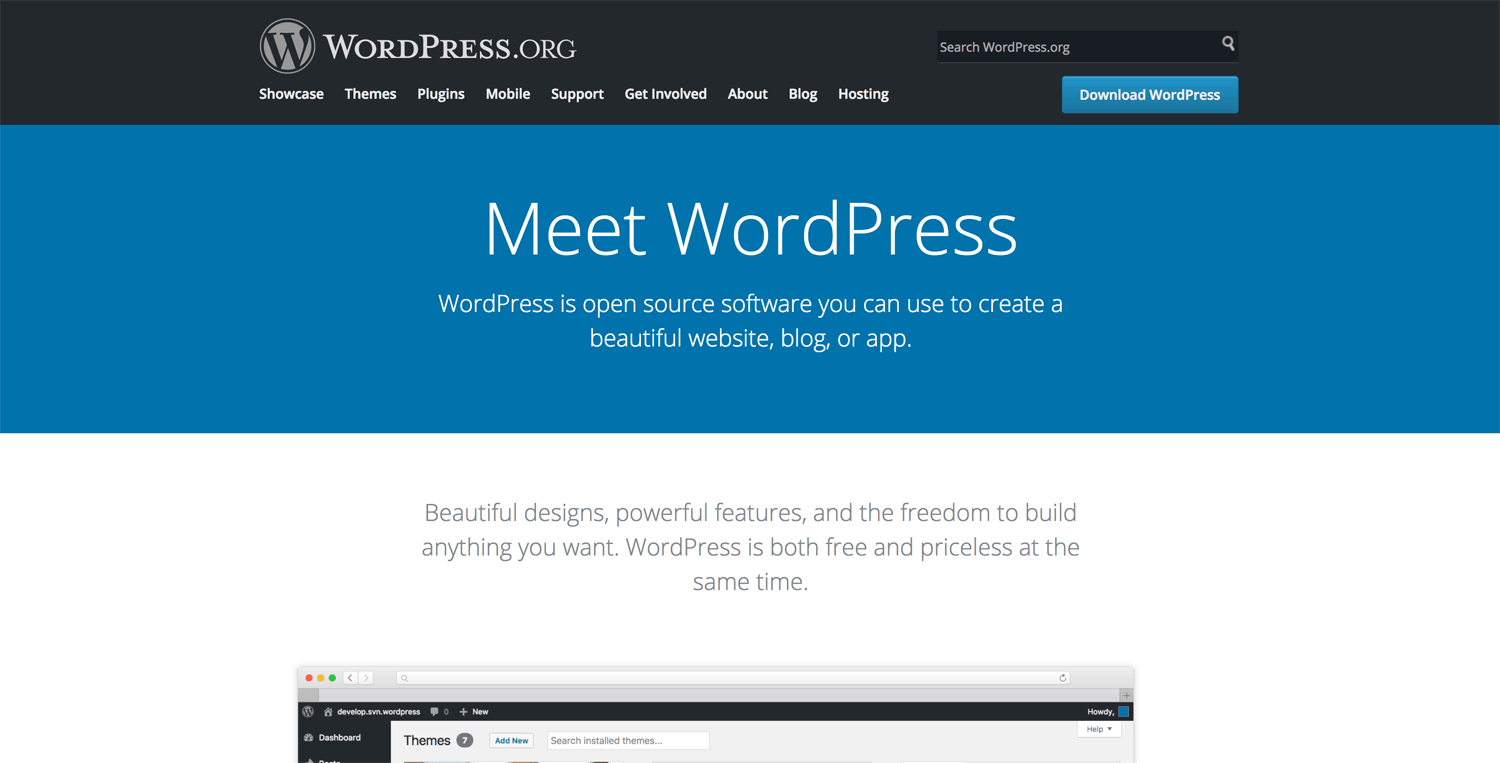This image is a detailed screenshot from the homepage of wordpress.org, showcasing the interface and design of this prominent content management system. The software is highlighted as open-source and free, making it an accessible tool for creating webpages.

At the top of the image, the header features a black background. On the left side, the WordPress logo appears—a gray circle with a stylized, black letter "W" in the center, accompanied by the text "wordpress.org" in white. Below the header runs the main menu, also in white font, listing navigation items: "Showcase," "Themes," "Plugins," "Mobile," "Support," "Get Involved," "About," "Blog," and "Hosting."

On the right side of the header, there’s a blue rectangular button with "Download WordPress" written in white, situated directly above a search box set against the same dark background. The search box, outlined in gray, includes the prompt "search wordpress.org" and an accompanying search icon on the right.

Transitioning from the dark header, a bold blue section captures the eye with the text "Meet WordPress" in white font. Below this, a description reads, "WordPress is open source software you can use to create a beautiful website, blog, or app."

Following this, the background shifts to white, presenting the text in gray: "Beautiful designs, powerful features, and the freedom to build anything you want. WordPress is both free and priceless at the same time."

Further down, a small section of the WordPress dashboard interface is visible, specifically the top of the "Themes" page, giving a preview of the user experience when managing a website within the platform.